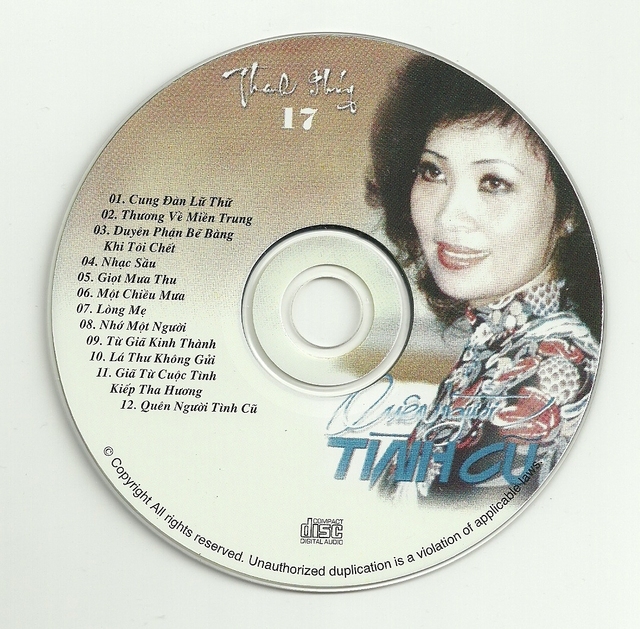The image features a small compact disc, approximately 4 to 5 inches in diameter, set against an almost white, very light gray background. In the center of the disc, a circular CD showcases an elaborate design. Along the left side, the numbers 0 to 12 are clearly marked, accompanied by a tracklist of 12 songs written in Vietnamese. At the top, an unreadable cursive in white is inscribed, followed by the number 17.

Dominating the right half of the CD is a vibrant image of an Asian woman, who appears to be the artist featured on the disc. She has black, outward-curled hair, thin black eyebrows, and heavy eyeliner accentuating her brown eyes. Her smiling face reveals the top row of her teeth, enhanced by thick lipstick. She is adorned in a high-necked floral blouse, rich with intricate patterns. Just beneath her image, her name is likely written in blue cursive and print, though it's illegible.

The bottom center of the disc is labeled "compact disc digital audio," and an important legal notice wraps around the lower edge, stating, "© copyright all rights reserved unauthorized duplication is a violation of applicable laws."